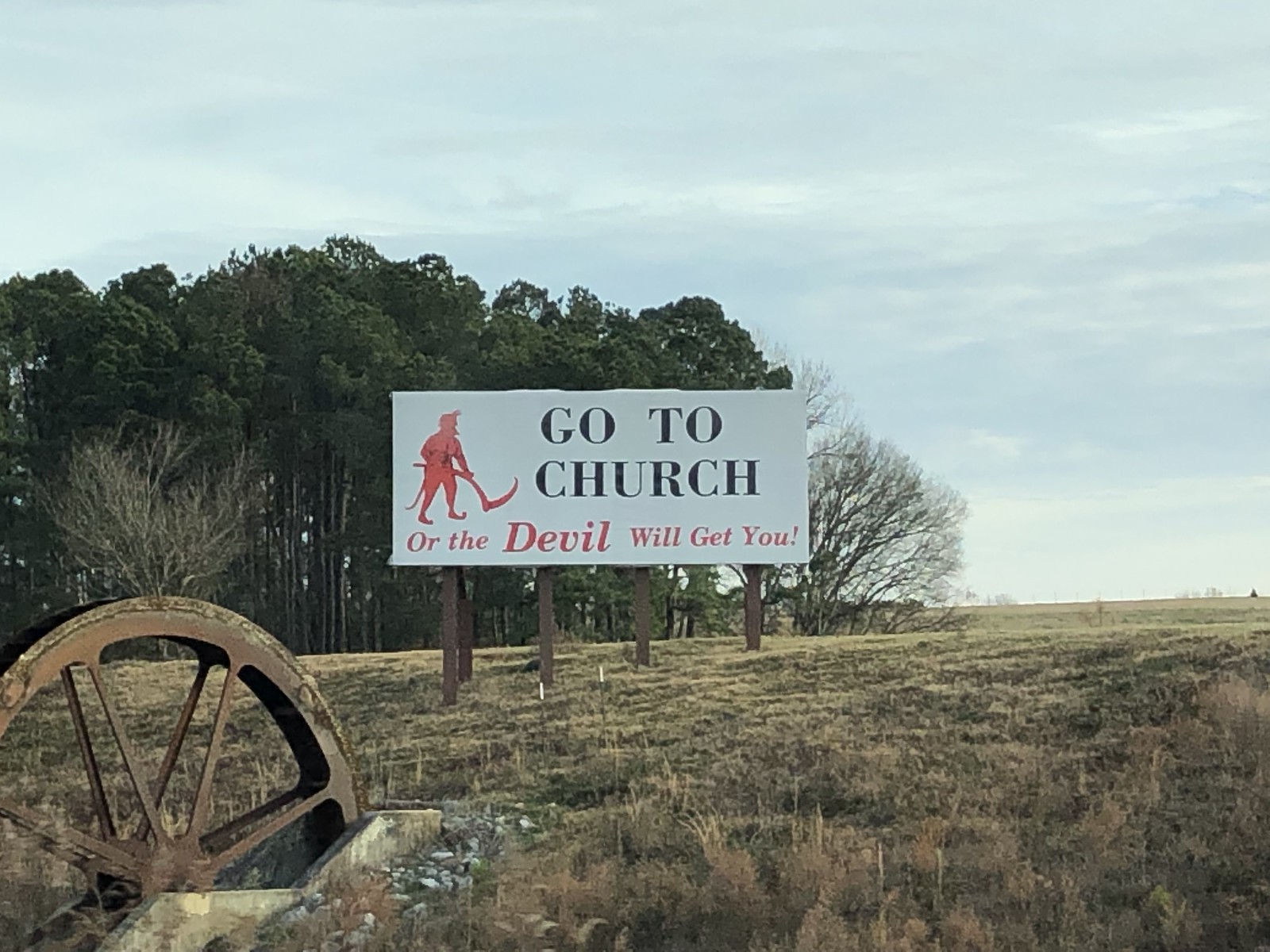The photograph depicts a striking roadside advertisement or billboard, mounted firmly on wooden poles. The rectangular white sign features an ominous black and red message: "Go to church or the devil will get you." The text is accompanied by an illustration of what appears to be the devil on the left-hand side, clutching a traditional scythe, evocative of the grim reaper poised to harvest souls that stray from the church. This kind of chilling advertisement is likely found in deeply religious regions of America, possibly the Bible Belt or the southern states, where church attendance is a cultural cornerstone.

The background of the image showcases a dense forest with very tall trees, some of which are bare and look lifeless—almost as if touched by decay or the harsh embrace of winter. The grass below the billboard and throughout the field is similarly desolate, appearing dry, burnt, or perhaps simply dormant for the season.

Adding to the eerie abandoned atmosphere, the sky overhead is a dull, muted blue, streaked with wispy white clouds. In the foreground, to the left, lies the weathered remnant of what once was a mine shaft wheel, now rusted and abandoned. This rusted artifact speaks of a bygone era, hinting at the existence of an old mine nearby, long since silent and unused.